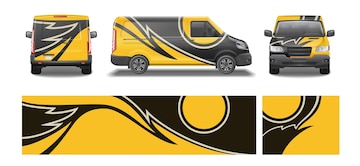The image displays a strikingly modern delivery van adorned in bold bumblebee-like colors of black and yellow. The detailed decoration spans the entire vehicle, creating a dynamic and noticeable appearance. There are three distinct views of the van: the back, side, and front. The rear view showcases an eye-catching zigzag pattern, partly yellow and partly black, with a white zigzag outlined on the black section. The side view highlights the predominantly yellow body featuring a white outline resembling a wing or a lightning bolt running the full length of the van's black center. This motif continues seamlessly over the roof. The front view reveals a split design, with the left side in yellow and the right side in black, featuring black side mirrors, a black windshield, a black grill, and white headlights. Accompanying these views, a close-up image displays intricate swirls and circles outlined in white on the black sections, accentuating the vivid contrast against the yellow background. The van's bold graphics and vivid colors make it an eye-catching and dynamic vehicle, though its size remains uncertain, potentially being a miniature model or a full-sized van.